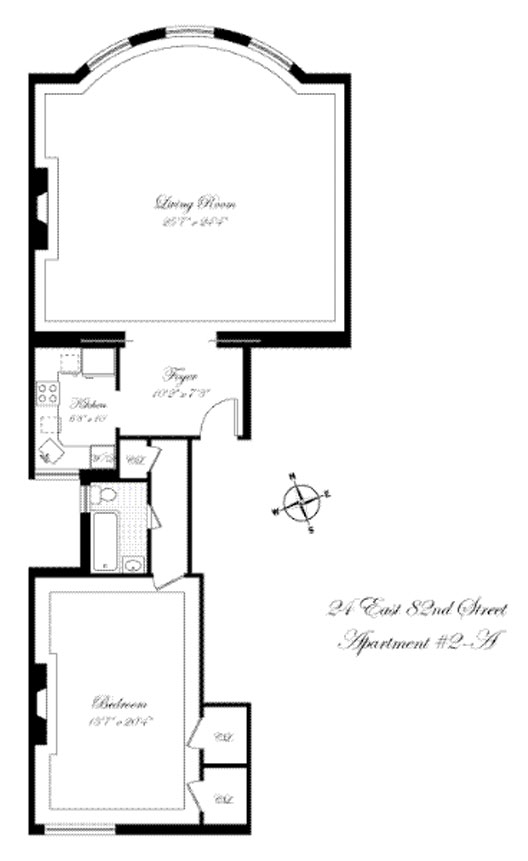This image is a black-and-white floor plan of an apartment located at 24 East 82nd Street, Apartment 2-A. The layout features clearly outlined rooms with accompanying, albeit difficult-to-read, descriptions in white. Despite the small and challenging text, the plan reveals a spacious living room, a foyer, a fully equipped kitchen, a compact bathroom, and a bedroom with an adjacent closet, indicative of a one-bedroom apartment. While no pricing information or city details are provided, the dimensions of each room are meticulously included, adding context to the size and potential layout of the space. The overall design is stark and minimal, serving primarily to give a general understanding of the apartment’s structure and flow.